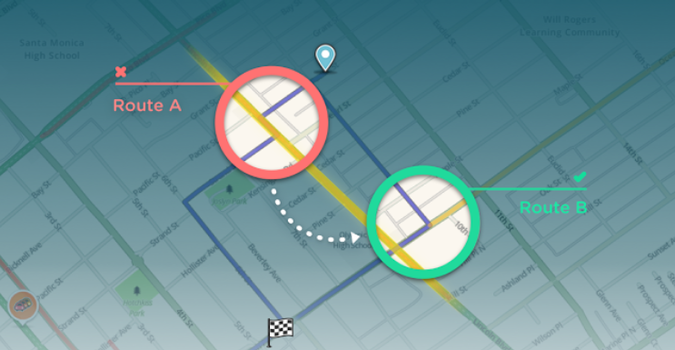This image is a partial screenshot of a navigation or mapping application, similar to Google Maps. The background of the image portrays a city map in a simplified format, with colored lines representing different routes. Thick green lines and a thicker blue line likely denote separate routes, with the blue line indicating a primary direction. A transparent, dark blue gradient overlay covers most of the map, which fades from dark at the top to lighter at the bottom.

In the center of the image, a red circle highlights a specific portion of the map, free from the blue gradient, for clear viewing. A line extends from this red circle, terminating in an 'X' symbol and labeled "Route A." Nearby, toward the top right, there's a location pin icon. To the lower right of this red circle, there's an identical-sized sea green circle focusing on another map segment, also clearly visible without the blue overlay. From this sea green circle, a line extends outwards with a check mark above it and labeled "Route B."

At the bottom center of the image, a checkered flag symbol is displayed, indicating a destination point. Some street names are visible, including "Ashland," "Wilson," "P.I.," and "4th Street." Additionally, an orange icon depicting a car is situated at a specific location on the map. The overall visual and functional features closely resemble those found in Google Maps.